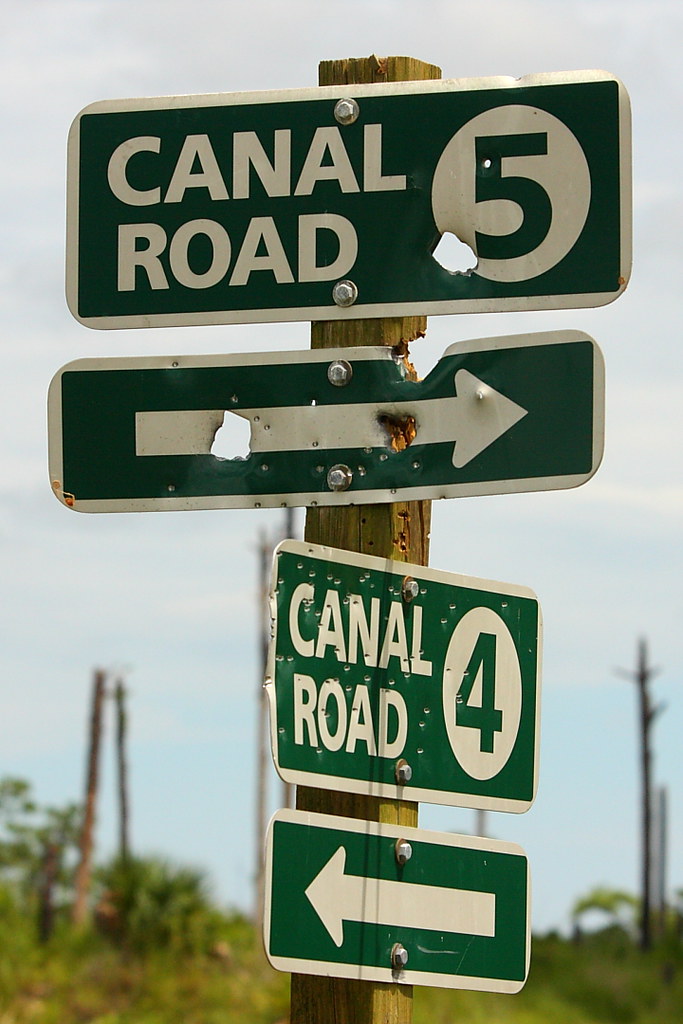The image depicts a cluster of green road signs affixed to a wooden post with silver fasteners. The top sign reads "Canal Road" in white text, featuring the number 5 within a white circle that has a large bullet hole in its bottom left area. Directly below, there is a sign with a white arrow pointing to the right, also showing signs of damage with chips, dents, and bullet holes near the end of the arrow, as well as an orange and black area towards the tip. Further down, slightly perpendicular, is another sign identical to the first but indicating "Canal Road 4," also marred with puncture holes. Finally, at the very bottom, there's another sign with a white arrow pointing to the left. All signs are outlined in white, consistent in design and uniformly displaying white text and arrows.